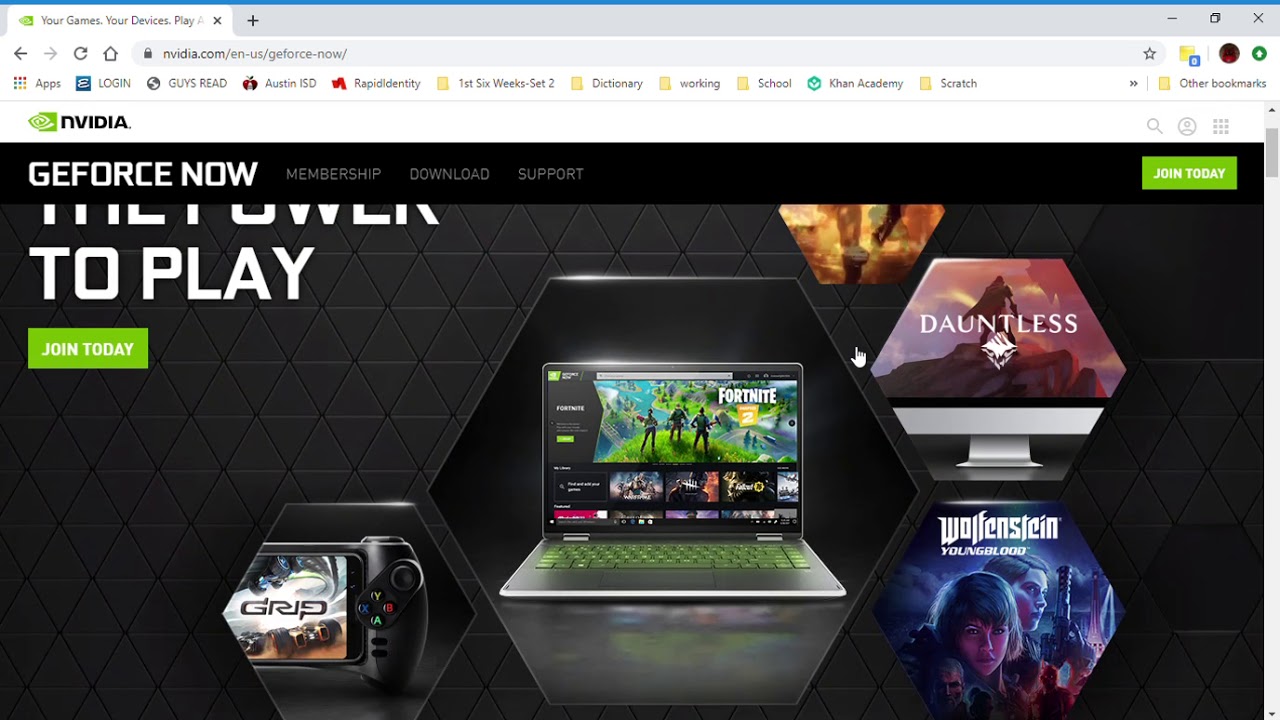The image is a detailed screenshot of an NVIDIA website, featuring a visually rich design. The background is an almost solid, very dark gray, overlaid with subtle diamond-shaped patterns for texture. At the top of the page, there's a narrow white banner displaying the NVIDIA logo. The logo consists of the word "NVIDIA" in black capital letters with the first 'N' styled to resemble lowercase, accompanied by a lime green square featuring a distinctive crescent shape.

Prominently displayed on the lower left-hand side is a bold headline, "GEFORCE NOW," written in white capital letters. Below this headline, the partial text "... TO PLAY" is visible, although the word above it is obscured by a black border.

The central focus of the image is a pentagon-shaped photograph showcasing a laptop with a silver-gray surface. The keyboard keys of the laptop are backlit in a matching lime green. The screen displays vivid imagery from the video game Fortnite. Flanking the central image are additional pentagon-shaped photos on both sides. On the right are images for the games Dauntless and Wolfenstein, while on the left, there's an image for the game Grip. Each image enhances the overall theme, creating an engaging and visually cohesive layout.